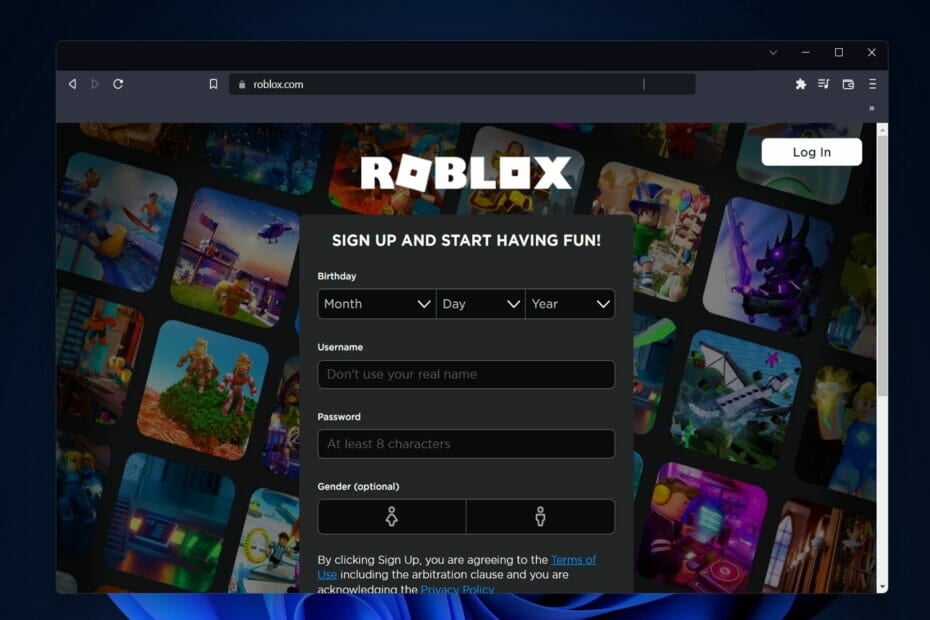A screenshot featuring a blue background depicts a sign-up page for "ROBLOX," with the logo prominently displayed at the top. The "O" in ROBLOX is creatively designed as a block tilted to the right. Below the logo are navigation symbols, including a left arrow, a right arrow (which is notably a lighter gray), a refresh button, and a bookmark icon. There is also a puzzle piece icon, three or four small rectangles, a music note, a square, a hamburger menu icon, and a login button within a white rectangle.

The main content of the screenshot includes a sign-up prompt encouraging users to "Sign up and start having fun." There is a section for entering a birthday with three black rectangles labeled "Month," "Day," and "Year." Directly beneath this, users are prompted to create a username and password, each with a corresponding text box. An optional field for selecting gender features two black rectangles: one with an icon of a woman in a dress and the other with an icon of a man in pants. Additionally, there is a "Sign Up" button in a grey square.